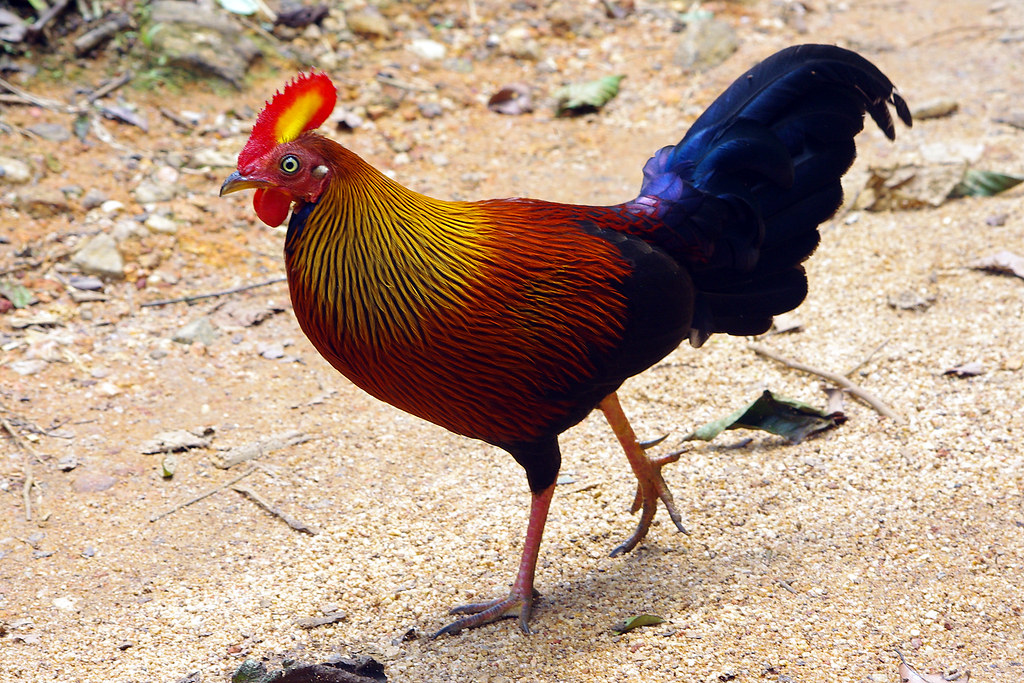The image captures a vibrant and healthy male cockerel or rooster, characterized by its splendid and multi-hued plumage. The bird is walking on a sandy path, surrounded by twigs, sticks, and rocks, against a backdrop featuring some greenery. The cockerel faces left, providing a clear side view as it struts confidently. Its head is adorned with a striking, colorful crest that is bright red on the outside and yellow in the center, complemented by vivid blue-green eyes. Beneath its gray beak, two red wattles dangle gracefully. The feathers on its head are small, shifting into yellow as they move down its neck. As the feathers progress down its body, they gradate into a vibrant rust-orange before transitioning into a dark blue-gray or nearly black shade along the back and tail. The magnificent tail feathers exhibit hues ranging from light blue to dark indigo, enhancing its regal appearance. The rooster’s legs are pink, ending in three front toes and a back claw, each leg featuring a prominent and sharp spur, indicative of its gender and role. Overall, the rooster emanates both elegance and health.